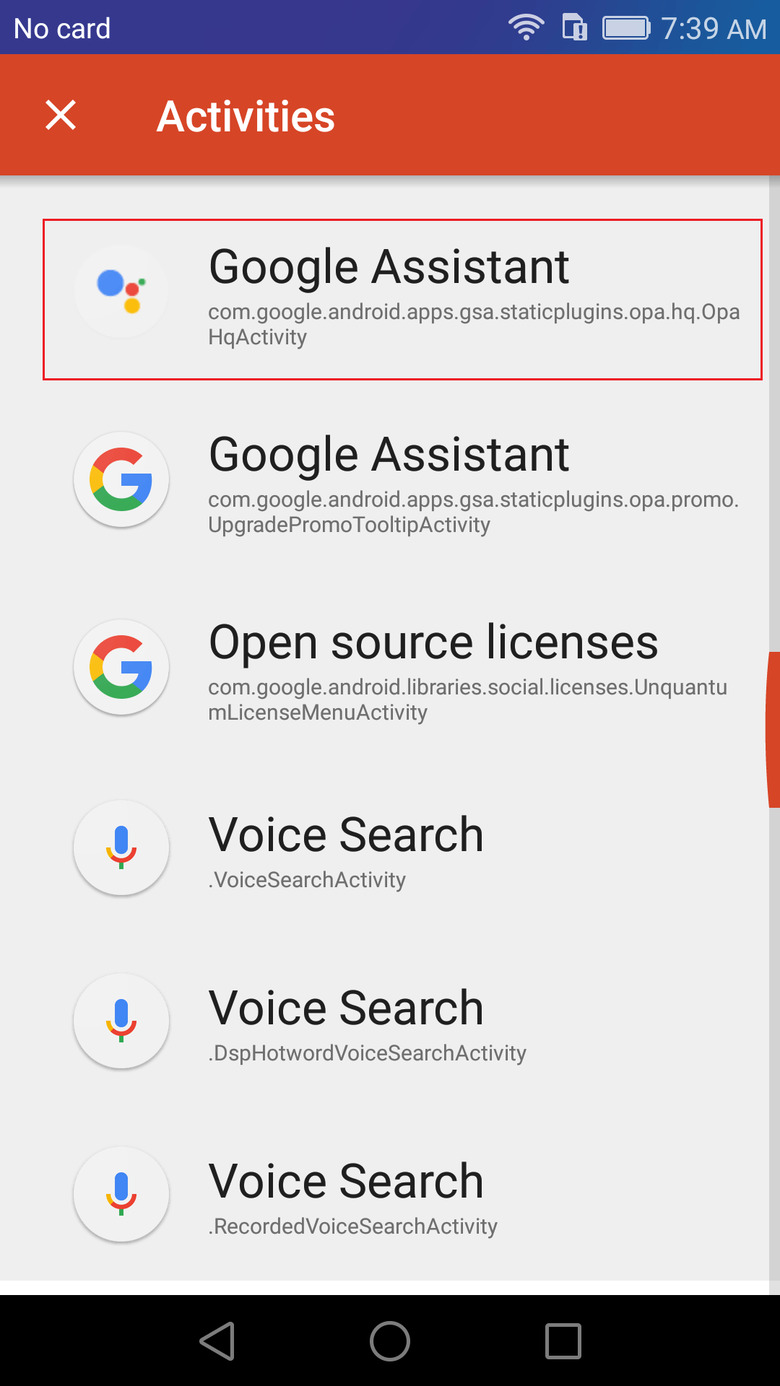The image displays several elements, each with specific details and formatting:

1. A portion of the image is devoid of any cards, timestamped at 7:39 AM, placed on a blue line.
   
2. Another section, highlighted by a red line, contains various activities marked with an 'X'. Within this section:
   - There is a reference to Google Assistant, specifically noted as `com.google.android.apps.gsa.staticplugins.opa.hq.OHQActivity`. Both "O," "H," and "A" in "OHQActivity" are capitalized. This entire reference is enclosed within a red rectangle.
   - Another mention of Google Assistant, `com.google.android.apps.gsa.staticplugins.opa.promo.upgrade.ToTipActivity`, includes capitalized letters "U," "P," "T," and "A" in their respective words.

3. Additionally, the image specifies open source licenses, indicated as `com.google.android.libraries.social.licenses.UNQANTUM.License.MenuActivity`, where "L," "M," and "A" are capitalized in "License," "Menu," and "Activity," respectively.

These elements are clearly demarcated and highlighted with appropriate lines and rectangles, ensuring ease of identification and readability.